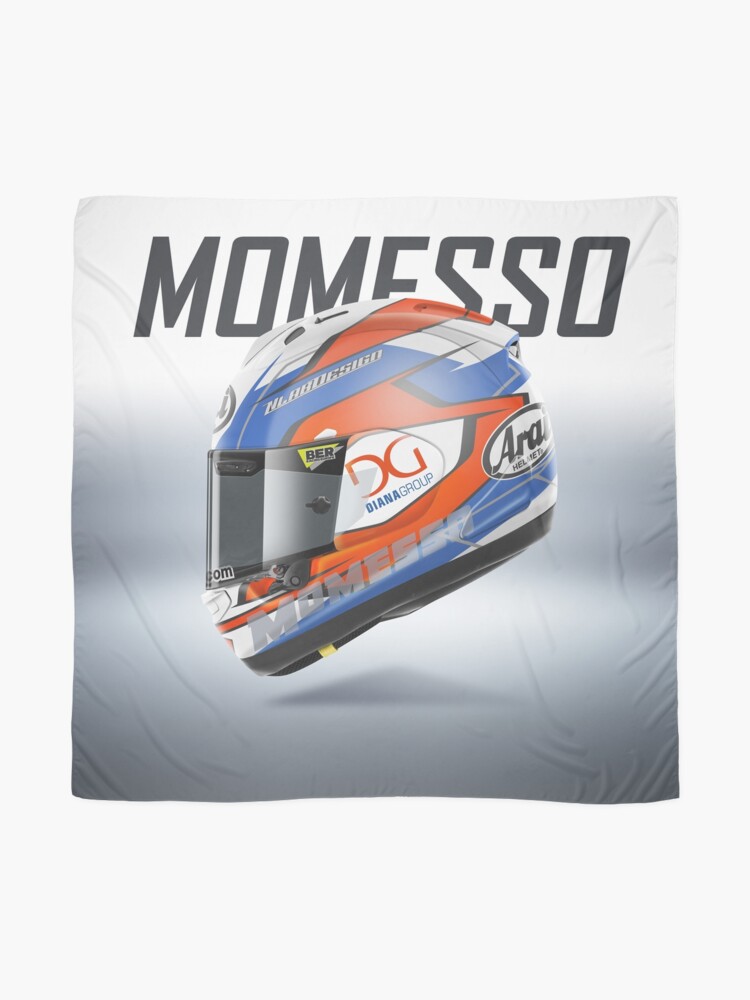The image portrays a sophisticated magazine advertisement featuring a high-performance racing helmet against a stylish three-tone background that transitions from white at the top through steel gray and into a darker variation of gray at the bottom. Across the top, large, bold black lettering spells out "Momesso." The centerpiece of the image is a close-up of the helmet, which is depicted with intricate details and a polished finish.

The helmet exhibits a striking color scheme of blue, red, and white. The crown of the helmet is primarily white, accentuated with red and blue stripes that cascade along its sides. The front visor, which is smoky gray and in the down position, contributes to the helmet's sleek and aerodynamic design.

Notable are the sponsorship decals adorning the helmet. On the right side towards the back, there is a white oval with the letters "A-R-A" printed in black. The left side features a white background displaying the letters "D" and "G" in black, likely part of the branding from the Diana Group, as indicated by additional text in blue below it.

The background, seemingly made of fabric, adds a textured depth to the image, with visible wrinkles suggesting materiality and craftsmanship. This juxtaposition of a high-tech helmet against a soft fabric backdrop makes for an eye-catching and tactile visual, enhancing the overall appeal and narrative of the advertisement.